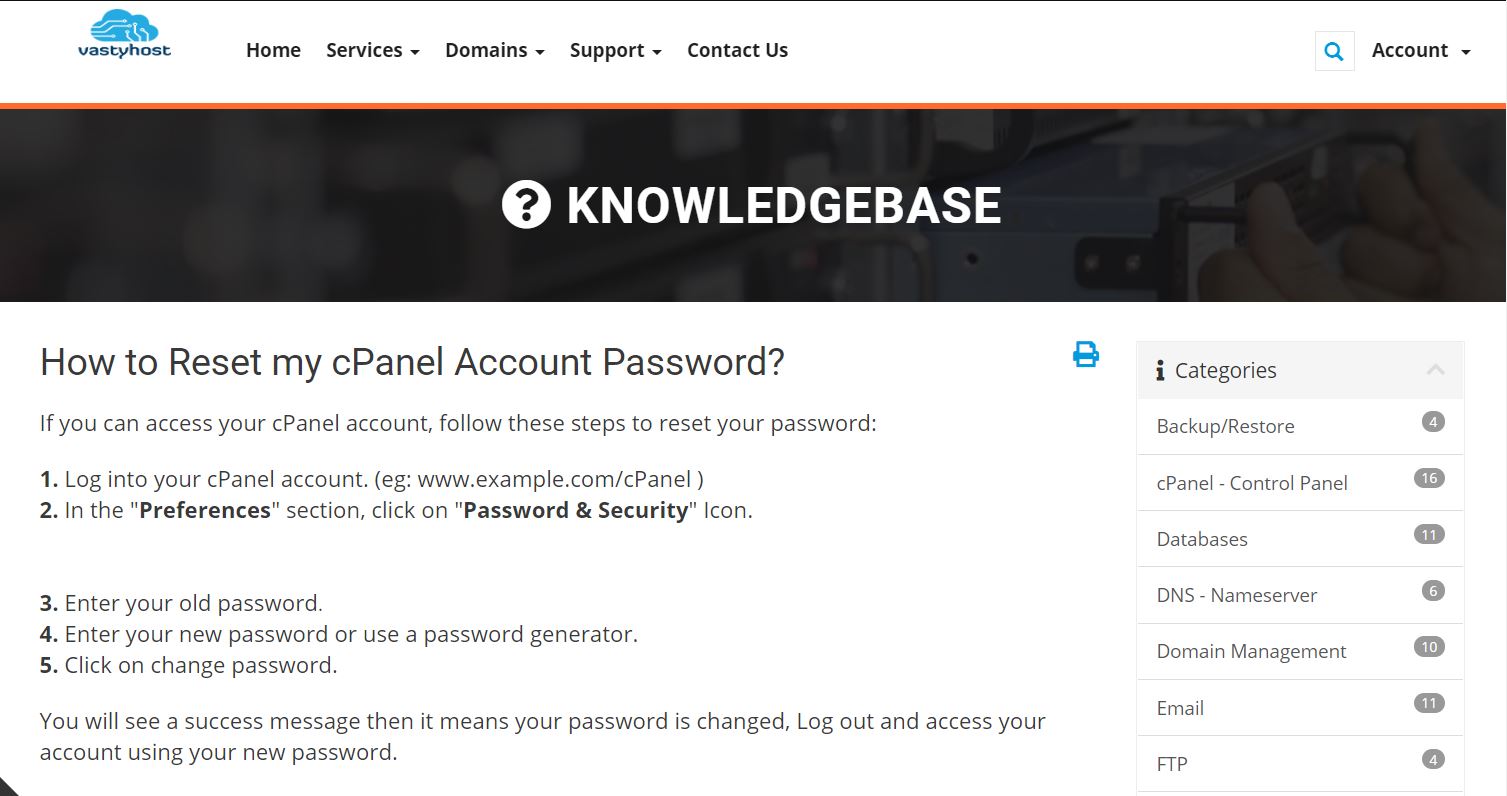The image is a detailed screenshot of a website interface for Vasti Host. At the top of the page, there is a horizontal navigation bar featuring various tabs labeled: Home, Services, Domains, Support, and Contact Us. To the far right of the navigation bar, there is a blue magnifying glass icon indicating the search function, followed by an "Account" link. The name of the company, "Vasti Host," is prominently displayed in the top-right corner of the screenshot.

Below the navigation bar, the title of the current page is "Knowledge Base." On the left side of the page, there is a specific article titled "How to Reset My cPanel Account Password," providing a step-by-step guide for users. The instructions read: "If you can access your cPanel account, follow these steps to reset your password. Login to the account. In the Preferences section, click on Password and Security. Enter your old password followed by your new password, or use a password generator to create a new password and then confirm the change."